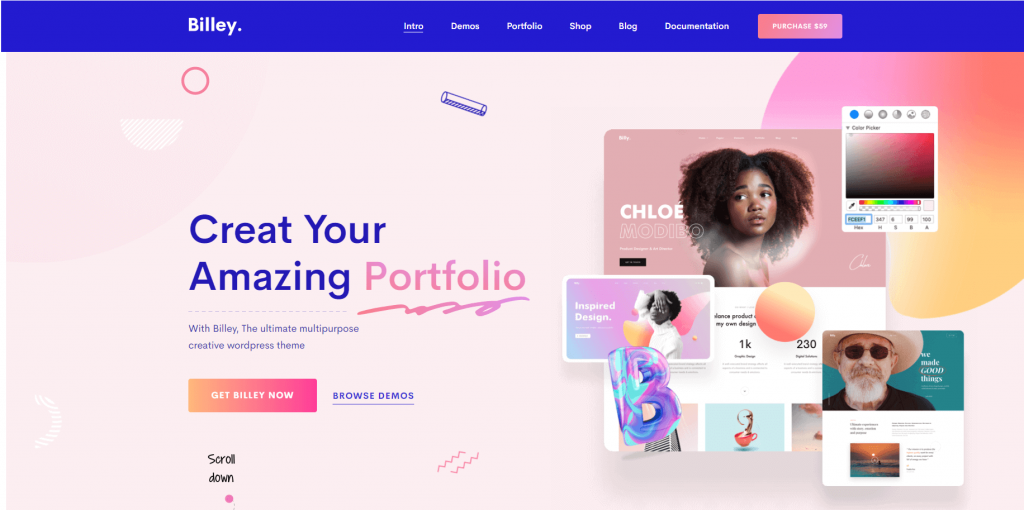This is a detailed screenshot of a web page titled "Billy." The header section features a blue background with the word "Billy" written in white on the left-hand side. Adjacent to this, the menu strip displays several navigation links also in white. There's a prominent pink button with white text, but the text is illegible due to poor contrast with the background.

The main section of the page has a light pink backdrop adorned with iridescent bubbles, creating a visually appealing effect. Overlaying this background, a multitude of pictures are layered in a somewhat chaotic manner. Text on both the left and right sides of the page reads "CREAT your amazing portfolio," with "Create" noticeably misspelled as "CREAT." Below this text, there's a call-to-action phrase "Get Billy Now," accompanied by a button that features a gradient from orange to pink.